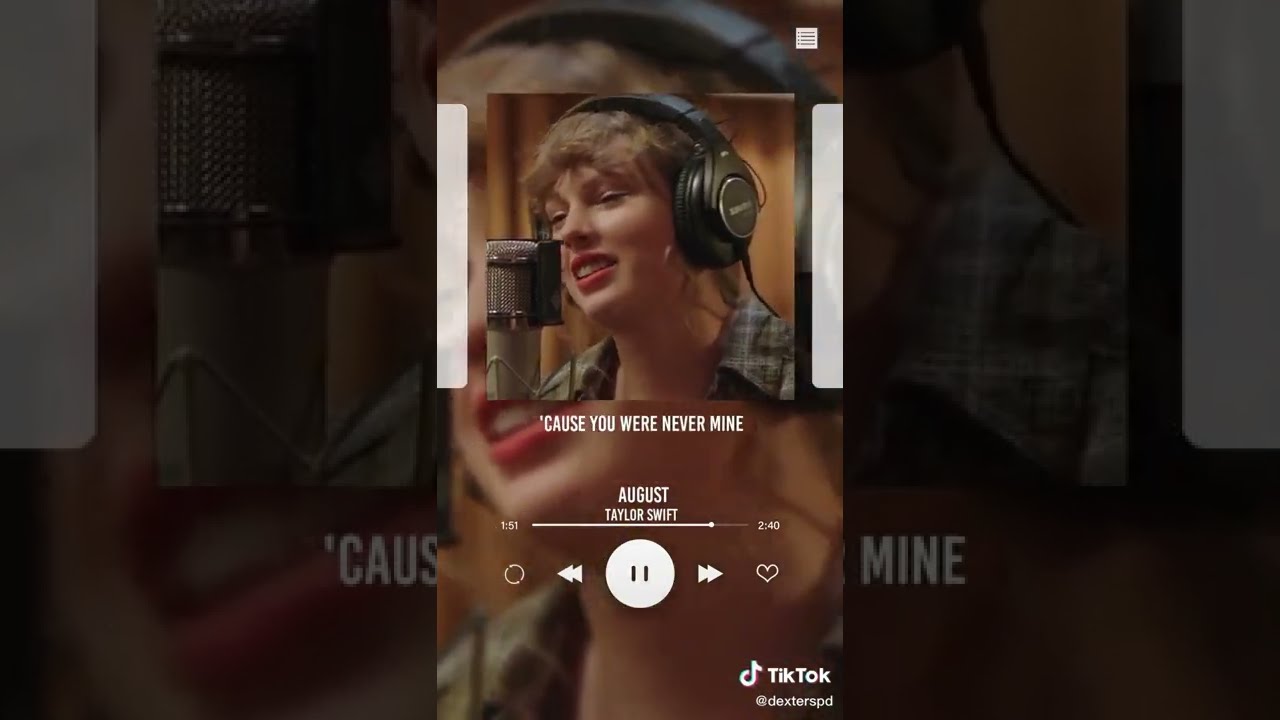In the screenshot of a TikTok video, Taylor Swift is at the center, wearing big silver and black headphones over her short hair, with her hair tied back. She is dressed in a plaid collared shirt and has red lipstick. Taylor is standing in front of a microphone, appearing to record in a studio setting. The screen displays the caption, "'Cause you were never mine," followed by "August," and then "Taylor Swift." A progress bar below the caption indicates that the song is at 1:51 out of 2:40 minutes. Control buttons for pause, rewind, fast-forward, repeat, and like are also present. The narrower image fits within the phone screen shape, while the background is a blurred, stretched version of the same image, giving the appearance of a double image. The TikTok logo is visible in the bottom-right corner, noting the user as Dexter SPD.